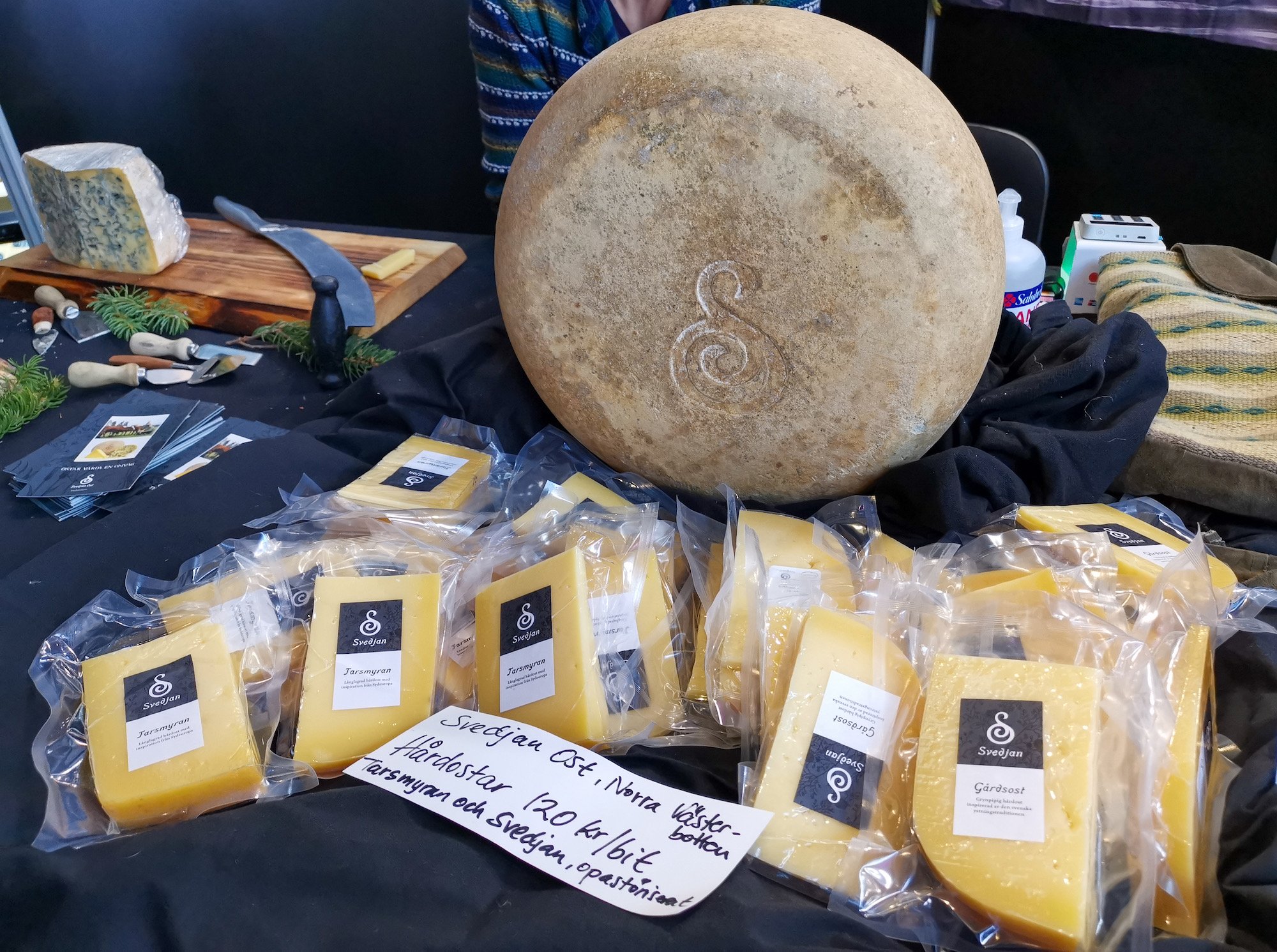A detailed display of cheese is set up on a navy-blue table at a bustling convention. Dominating the scene is a large, tan-colored, aged wheel of cheese prominently positioned at the center of the table. In front of the wheel are multiple packaged cheeses labeled "GARDOST" and "SVEDJAM," each featuring an elegant S-shaped logo. To the left, a wooden cutting board showcases another type of cheese, accompanied by a large knife positioned next to it, ready for slicing. Adding a splash of color to the setup, a striped shirt in white, green, blue, and yellow can be seen partially behind the wheel of cheese, though the person wearing it is cropped out of the frame. The overall presentation exudes an artisanal and sophisticated vibe, characteristic of a high-end cheese exhibition.